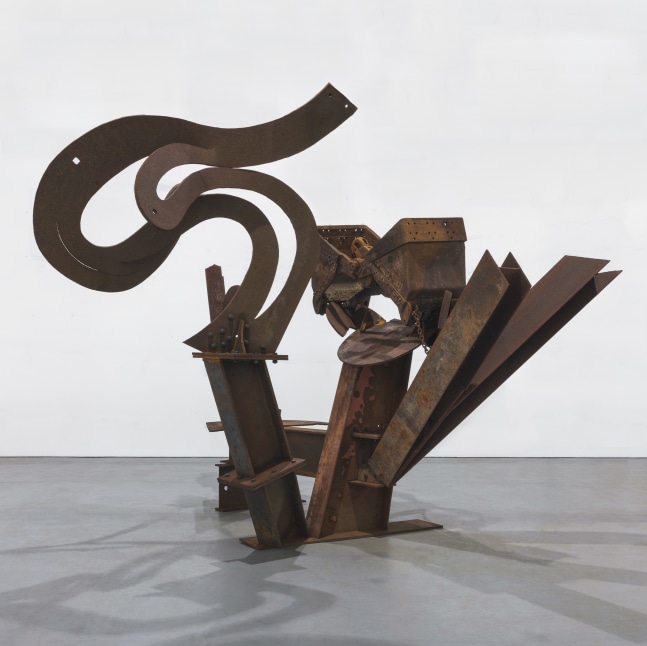This photo features an abstract metal sculpture situated presumably in an art gallery. The piece is composed of various rusty, brown steel components that intertwine and intersect in intricate formations. The base consists of steel girders that angle into a V-shape, with another V-shaped structure emerging from the right side. The sculpture integrates both straight and curved metal pieces, creating a dynamic visual balance. On the left side, there is a prominent curving, swirl that resembles an 'S,' contributing to its complex silhouette. Centrally positioned is a circular element atop the structure, joined by what appears to be a bowtie-like steel piece. The sculpture rests on a smooth, light gray floor with a plain, light gray wall serving as the backdrop. Despite the minimalist setting, the detailed and intricate metalwork suggests a blend of industrial and organic aesthetics. The composition, devoid of any text or additional elements, offers a focus solely on the sculpture, leaving its scale ambiguous and inviting contemplation.